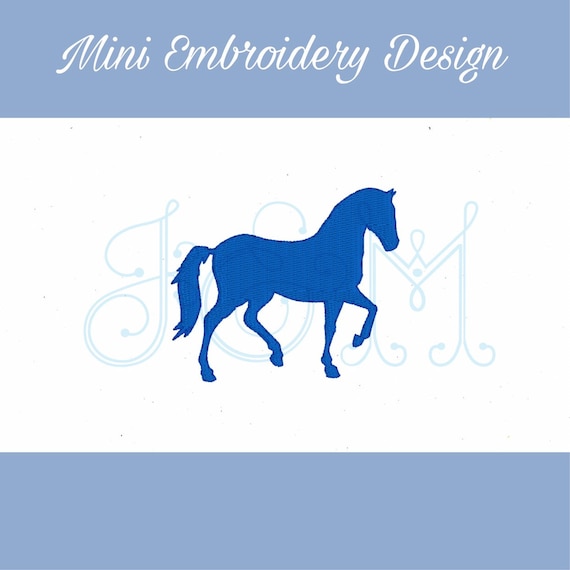This image titled "Mini Embroidery Design" appears similar to a flag and could be a product advertisement or a logo. It features two horizontal light blue rectangular strips at the top and bottom. The top strip contains cursive white text reading "Mini Embroidery Design." The central section of the image is predominantly white, serving as a contrasting backdrop for a blue silhouette of a horse located at the center. The horse, depicted in a darker blue, is facing to the right with its left front leg raised and its tail down. Behind the horse, in light blue and cursive font, are the letters "J M." The bottom blue strip is blank. The overall design suggests that this might be a logo for an embroidery company, with the horse possibly serving as the mascot.